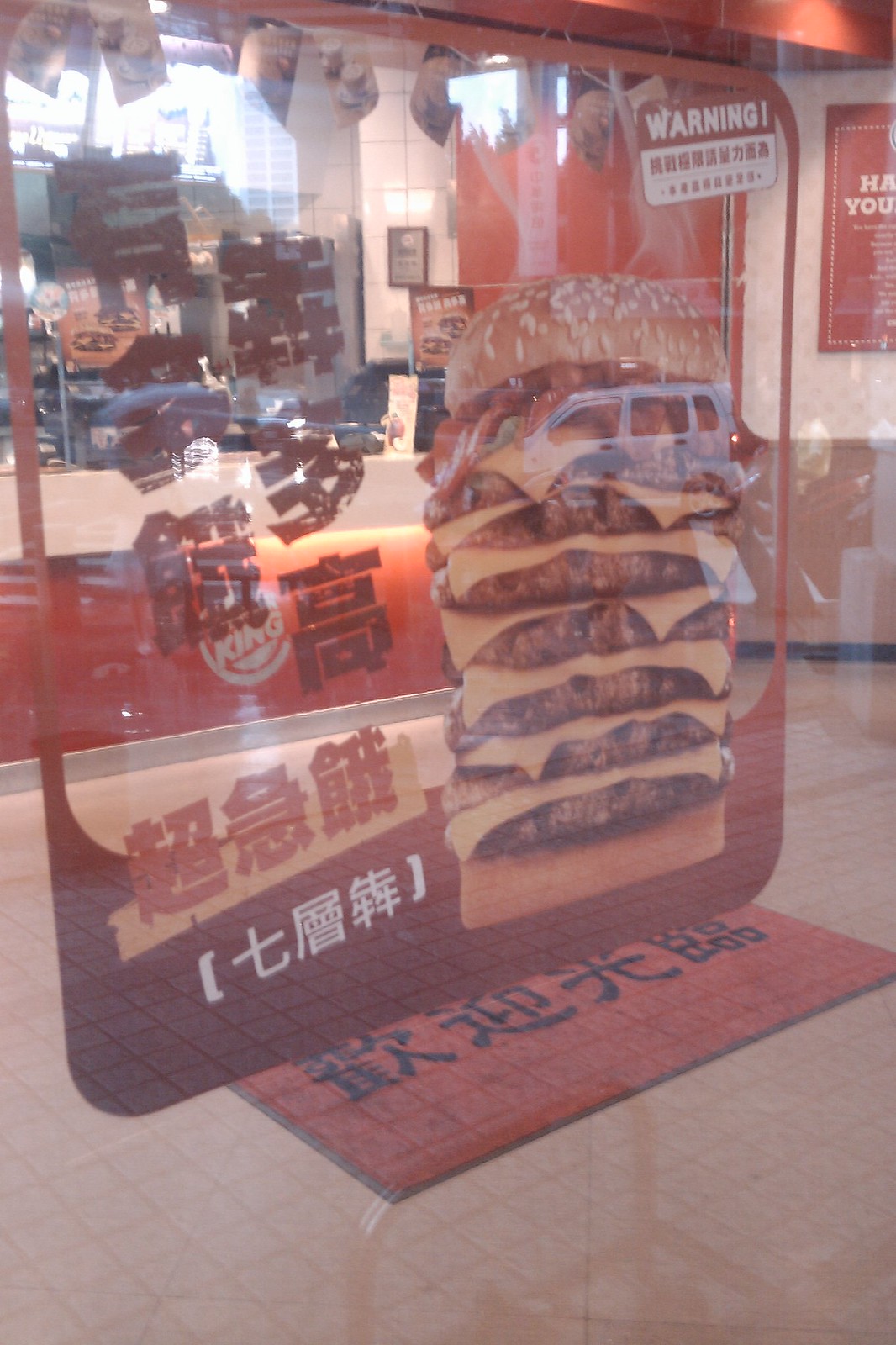The photograph, taken in an urban area in the Far East—likely China or Japan judging by the complex, vertical characters written on a red background—features the glass storefront of a Burger King. Prominently displayed on the window is a detailed graphic of a colossal, multi-tiered hamburger with at least six to eight beef patties, each separated by slices of cheese, and crowned with crispy bacon, lettuce, and a sesame seed bun. Next to this mouth-watering visual, the word "WARNING" is boldly printed in white on a red sign in the upper right corner, surrounded by additional Asian characters.

Inside the Burger King, visible through the reflections of vehicles including a white van on the street, is an orange and white counter bearing the Burger King logo. The interior features white tiled walls and gray kitchen machinery. A red mat with black Asian characters is noticeable on the tiled floor, adding to the authentic ambience. The image captures the inviting yet bustling atmosphere of this international fast-food outlet.